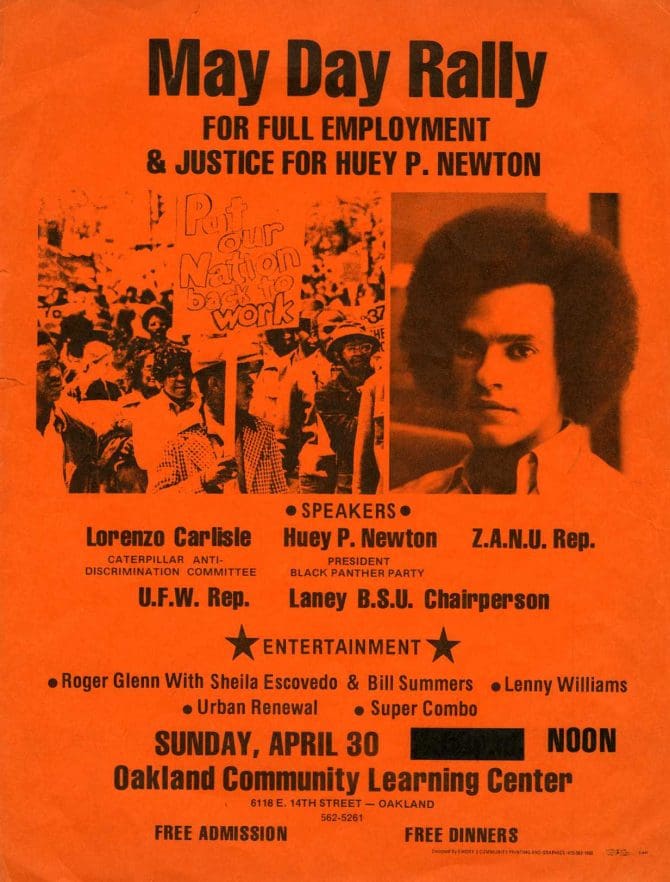This is a photograph of a vibrant orange flyer advertising a May Day Rally for Full Employment and Justice for Huey P. Newton. The flyer prominently features the heading "MAY DAY RALLY" in bold black text, followed by "FOR FULL EMPLOYMENT AND JUSTICE FOR HUEY P. NEWTON" in smaller all-cap letters. On the right side, there's a close-up photograph of Huey P. Newton, showcasing his afro and collared shirt. On the left side, there is an image depicting a diverse group of protesters holding signs, with one sign reading "Put Our Nation Back to Work."

The flyer lists several speakers, including Lorenzo Carlisle, Huey P. Newton, a ZANU representative, a UFW representative, and the Laney BSU chairperson. Under the "Entertainment" section, it highlights performances by Roger Glenn with Sheila Escovedo and Bill Summers, Lenny Williams, Urban Renewal, and Super Combo.

Details provided at the bottom of the flyer indicate that the rally will take place on Sunday, April 30th at noon, at the Oakland Community Learning Center, located at 6118 East 14th Street, Oakland. The event promises free admission and free dinners for attendees.